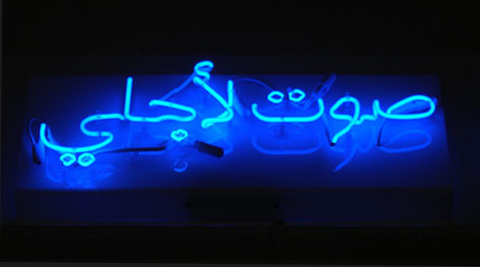The image features a glowing neon sign against a pitch-black backdrop, its electric blue light illuminating the surrounding darkness. The sign appears to be crafted in Arabic script, forming a single word that emits a bright blue aura, creating a striking contrast with the black field. From an angle looking slightly upward, the sign possibly advertises a club or bar. Near the center of the sign, a wide smiley face can be discerned, and scattered around the left side, there are additional circular neon shapes. The overall simplicity and the radiant glow of the Arabic lettering dominate the composition, making it a visually compelling and vibrant scene.